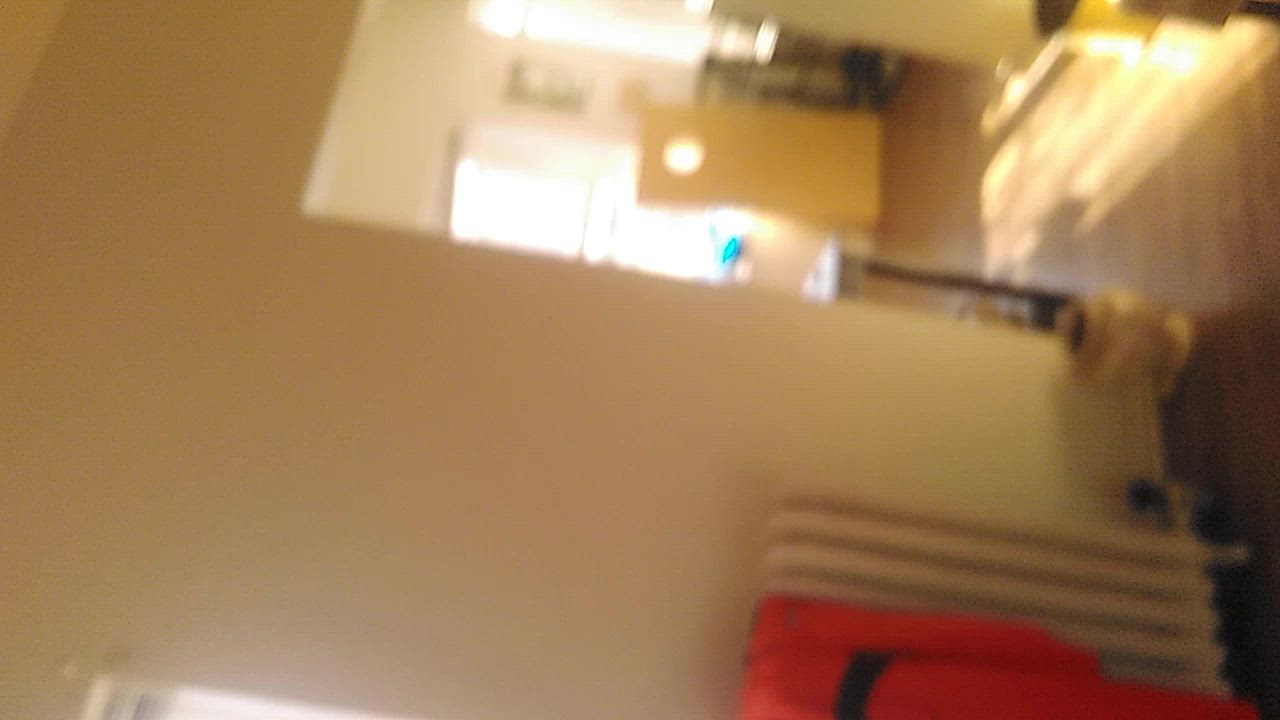The blurry photograph captures an interior room bathed in natural sunlight. The room features light-colored wooden floors in a lighter shade of brown, which are prominently visible. Against the white walls, a white radiator stands out, partially covered by what appears to be a red-orange article of clothing with a black stripe. Sunlight filters in through the windows, creating stark shadows from various objects onto the wooden floor. Near the radiator, a white pot sits slightly apart, adding to the room's minimalist decor.